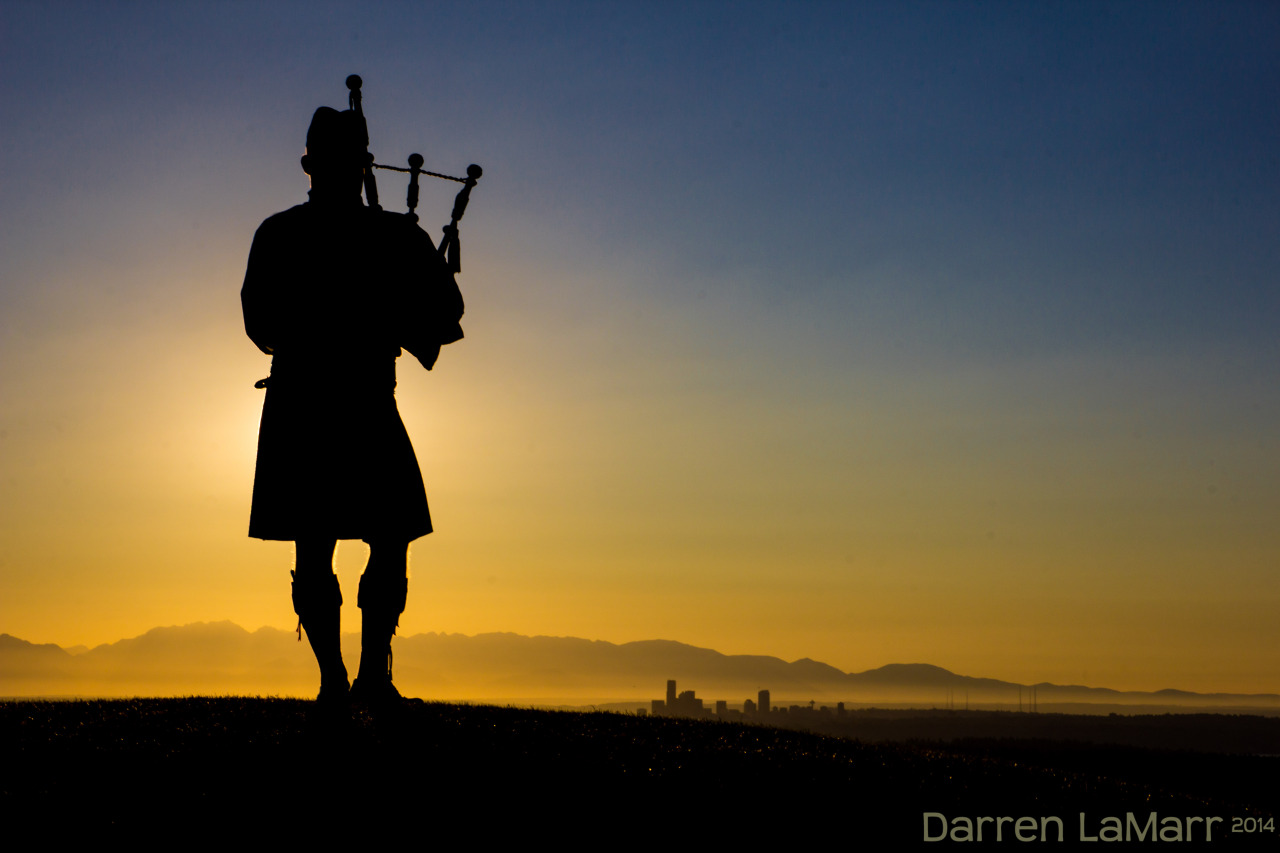In this striking landscape photo by Darren Lamar dated 2014, the silhouette of a lone bagpipe player stands on a black hilltop overlooking a distant town. The individual, dressed in a kilt and boots, is captured from a lower angle, making them appear large as they occupy the full height of the image. The sky above transitions from a dark blue at the top to a warm yellow near the horizon, with the bright sun directly behind the silhouetted figure, accentuating their blacked-out form. In the background, beyond the hill, a small town is visible, flanked by a range of subtle hills. The photograph captures a serene yet powerful moment, with the details creating a harmonious blend of natural beauty and cultural symbolism, underscored by the artist's signature and date in white text at the bottom right corner.